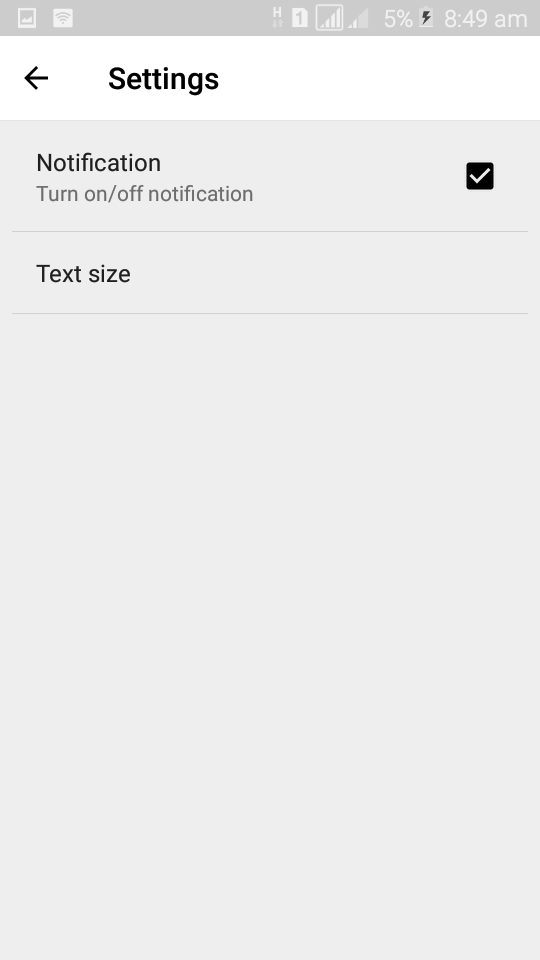A vertical screenshot of a phone settings screen, featuring multiple interface elements. At the top left corner, there's a photo icon followed by a Wi-Fi icon. To the right of the Wi-Fi icon is the letter "H," the number "1," a service symbol encapsulated in a square, another service symbol with 2 out of 5 bars, and "5%." Adjacent to these is a battery icon with a lightning symbol in the center. The time displayed is 8:49 AM, all of these indicators situated within a light gray status bar.

Below, there is a black-text back button and the word "Settings" in bold black text, highlighted by a white background. Underneath this header is a lighter gray section. The first subsection titled "Notification" includes an option to turn notifications on or off, which is currently enabled as evidenced by a white check mark within a black square. This section is demarcated by a horizontal line, followed by another option titled "Text Size," with a corresponding line below it.